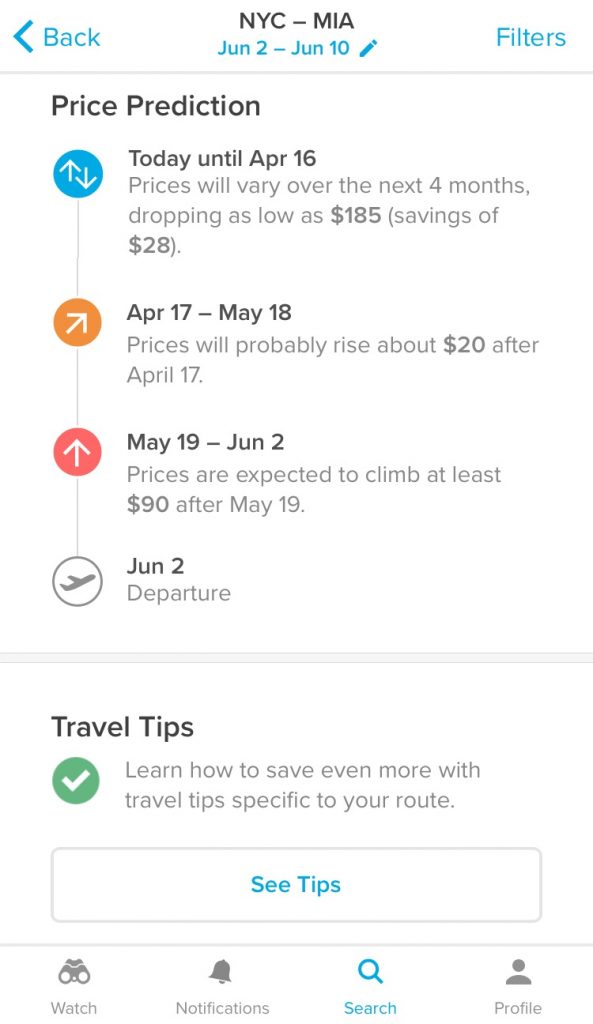This screenshot captures a mobile travel app displaying a flight itinerary from New York City to Miami, scheduled for June 2nd to June 10th. The app provides a price prediction feature, illustrating how ticket prices are expected to change from the current date up to the departure date. Specifically, it highlights three distinct date ranges with corresponding price trends: initial fluctuations, a probable rise in prices closer to the departure, and a significant price increase right before the flight. At the bottom of the screen, the app offers general travel tips. Additionally, it includes interactive buttons for setting fare alerts (Watch), enabling notifications, searching for flights, and accessing the user profile.